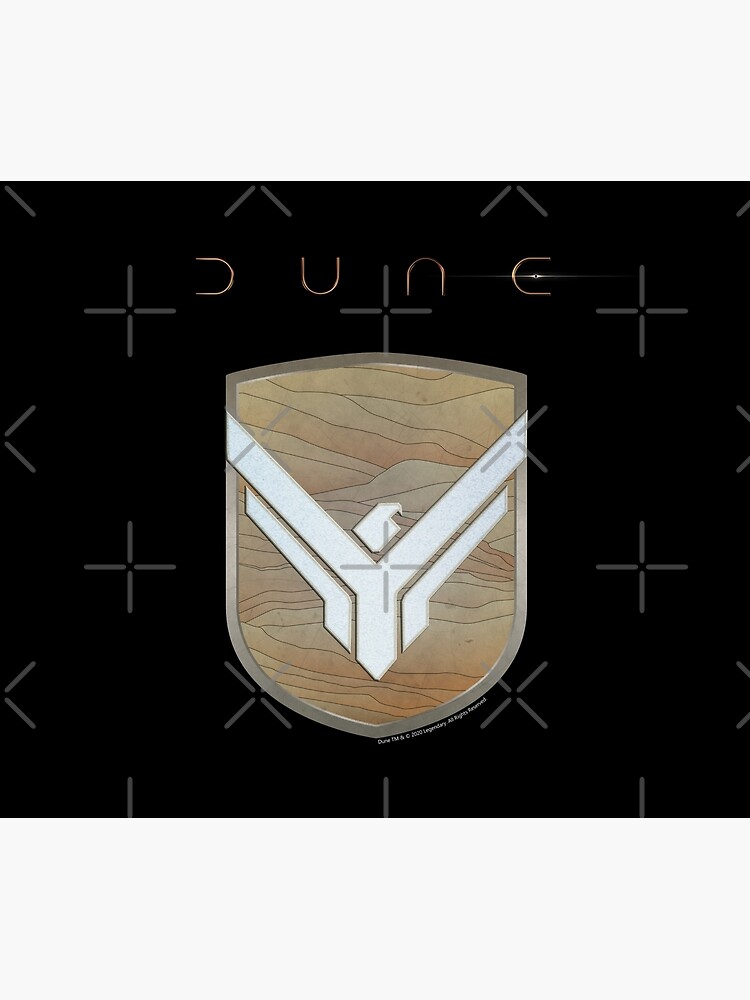The image is a perfectly square design with a black background. At the very top, in thin gold letters, it says "DUNE" with the "D" appearing as a half-letter missing its vertical stroke. Below this text, there is a central emblem resembling a shield or crest bordered in a metallic or gold-like color. The interior of the shield has a beige and reddish-beige background, resembling layered wood textures. In the center of the shield, there is a stylized depiction of an eagle or bird, crafted with white, tan, and gray colors, showing a body with extended wings to the left and right and a head turned to the right. Overlaying the black background are cream-colored plus and X symbols randomly spaced. The overall appearance suggests a blend of intricate details and simple design elements to create an emblematic logo.